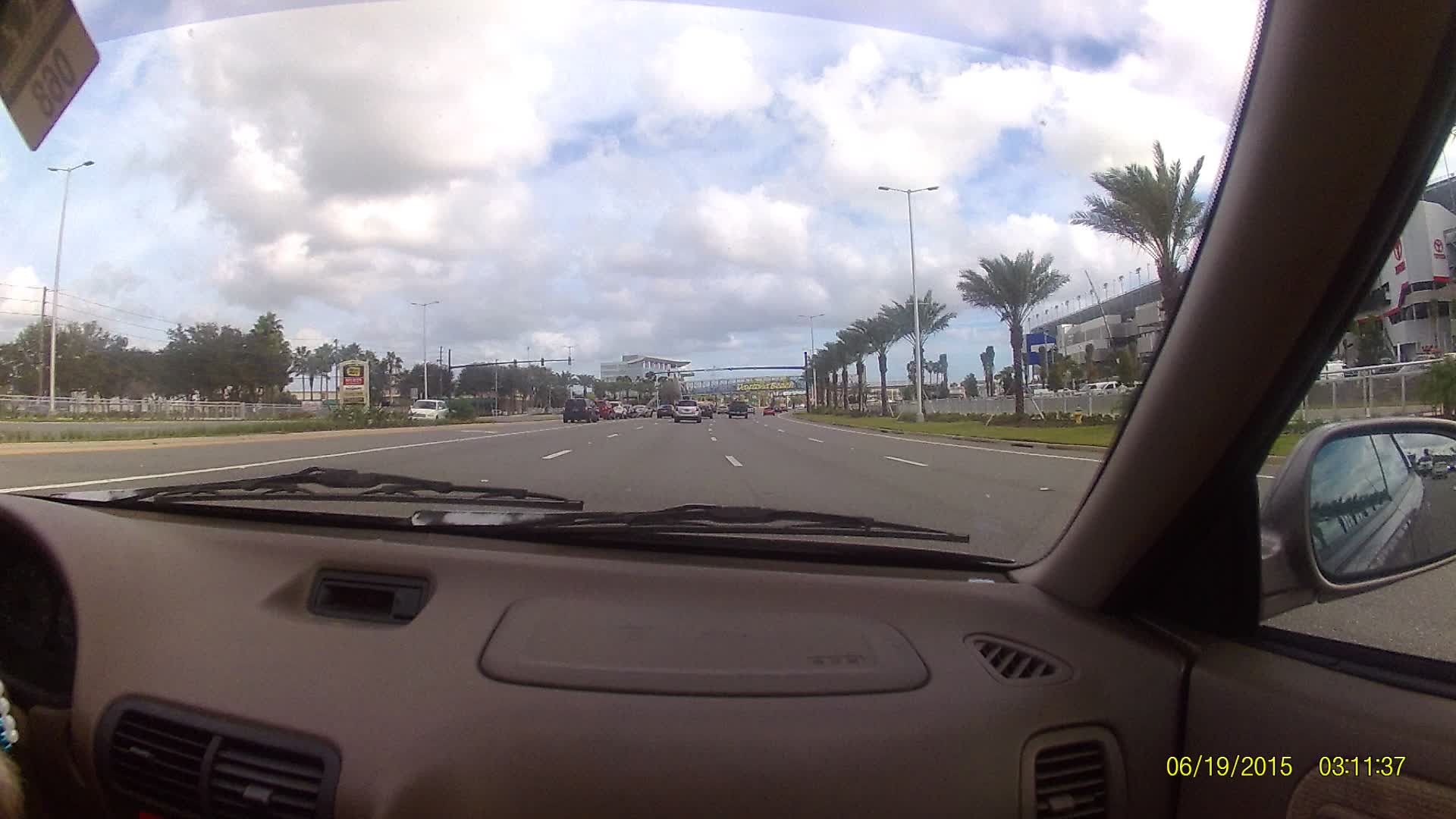The image is a detailed color photograph captured from the front passenger seat of a moving vehicle, looking through the windshield. It presents a landscape orientation of a bustling four-lane highway with an additional turning lane on the left, making it five lanes in total. The dashboard of the car is partially visible, featuring a couple of air vents on the right and two in the middle, as well as a gray rearview mirror with an object hanging from it, marked with the number "068." The photograph includes a yellow date and time stamp in the bottom right corner, reading "06/19/2015 03:11:37," suggesting it was taken in the mid-afternoon.

The road ahead shows several cars in the distance, hinting at a potential traffic buildup. On the right side, two lanes over, there is a green grass verge running alongside the highway with a steady row of palm trees and a building, possibly a car dealership, indicating a tropical area. Further up on this side, telephone poles and more commercial buildings come into view. On the left side of the image, dark green trees are visible, and a single car is seen traveling in the opposite direction. The sky above features thick clouds with patches of light blue, characteristic of a spring or summer day, adding a dynamic backdrop to the scene.